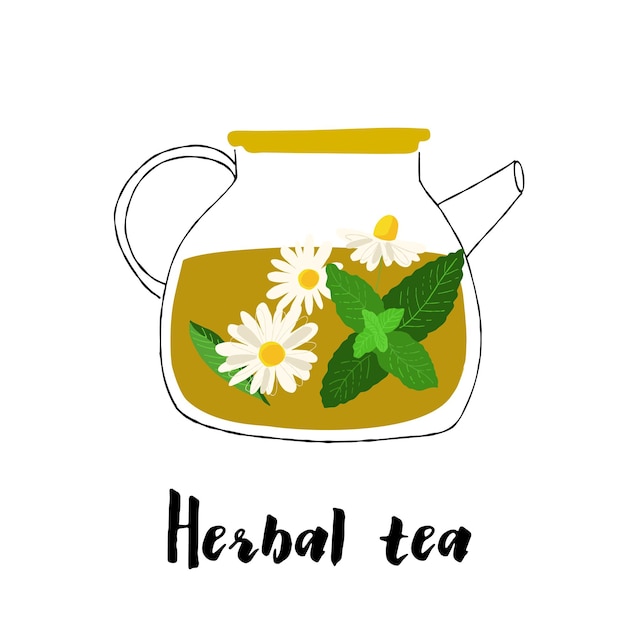This image features a hand-drawn illustration of a glass teapot against a white background. The teapot is transparent, allowing for a clear view of the contents inside. It is topped with a flat, deep yellow lid and has a handle and spout outlined in black, with white spaces in between the lines. Within the teapot, there is a green leaf situated at the bottom left. Also inside are three chamomile flowers, characterized by their white petals and yellow centers. Additionally, a sprig of mint is visible, featuring a distinct arrangement: two dark green leaves, two lighter green leaves placed in a cross-like fashion, and four smaller, even lighter green leaves also crossed. Beneath the teapot, in an elegant script, the words "herbal tea" are inscribed in black.